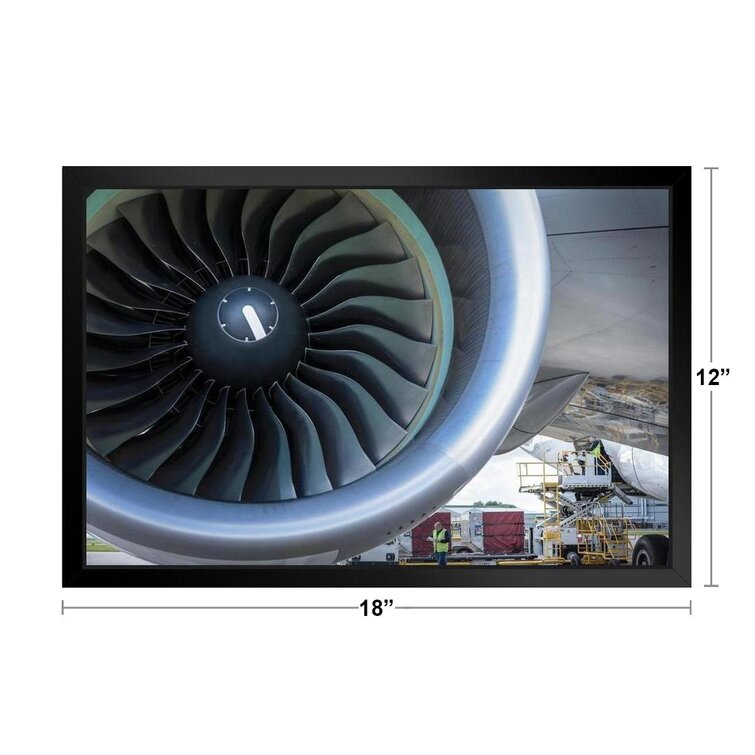This detailed color photograph presents a close-up view of a large airplane's propeller, taking up a significant portion of the image, primarily on the left side. The jet engine, cylindrical in nature with black internal components and a silver exterior, is prominently featured in roughly three-quarters of the frame, given the cut-off view. Beyond the propeller, on the right side of the image, a bustling scene of maintenance work unfolds. A worker in a green high-visibility vest appears to be engaged with tools and airplane equipment on a platform, possibly performing routine checks or repairs. Additional background details include a dark sky, a building with red sliding doors, and a yellow lift used for accessing elevated parts of the plane. The tarmac is partially visible beneath the aircraft's belly. The photograph is bordered by black lines with measurements indicating an 18-inch width and a 12-inch height, suggesting the dimensions of the image.